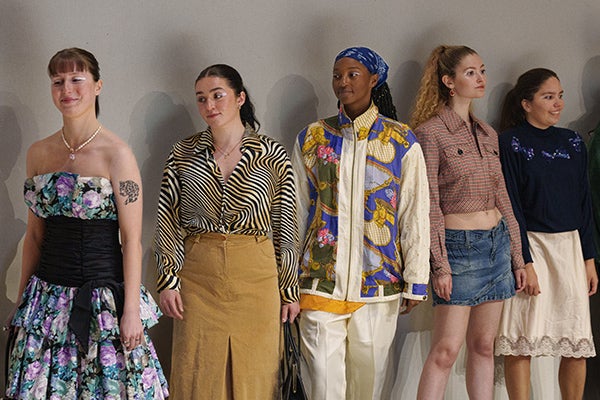This photograph features five young women standing in front of a gray wall, their shadows visible behind them, suggesting a light source from the front. From left to right, the first woman has dark brown hair pulled back into a ponytail and is wearing a floral-patterned sleeveless dress with a choker necklace and a black bow at the waist. She has a tattoo of a tiger on her left arm. The second woman, also with her hair in a ponytail, wears a zebra-striped blouse and a beige skirt with a slit. She has a small gold necklace. The middle woman, of African descent, has her hair back in a blue and white scarf. She is dressed in a blue-patterned beige jacket, a beige shirt peeking out, and matching beige pants. Next is a woman with blonde hair in a high ponytail, wearing a red midriff-baring top with a collar and pockets, paired with a short denim skirt. The final woman on the right has brown hair pulled back into a ponytail. She’s wearing a blue sweater with a white knee-length skirt. The group presents a diverse and vibrant display of fashion against a neutral backdrop.